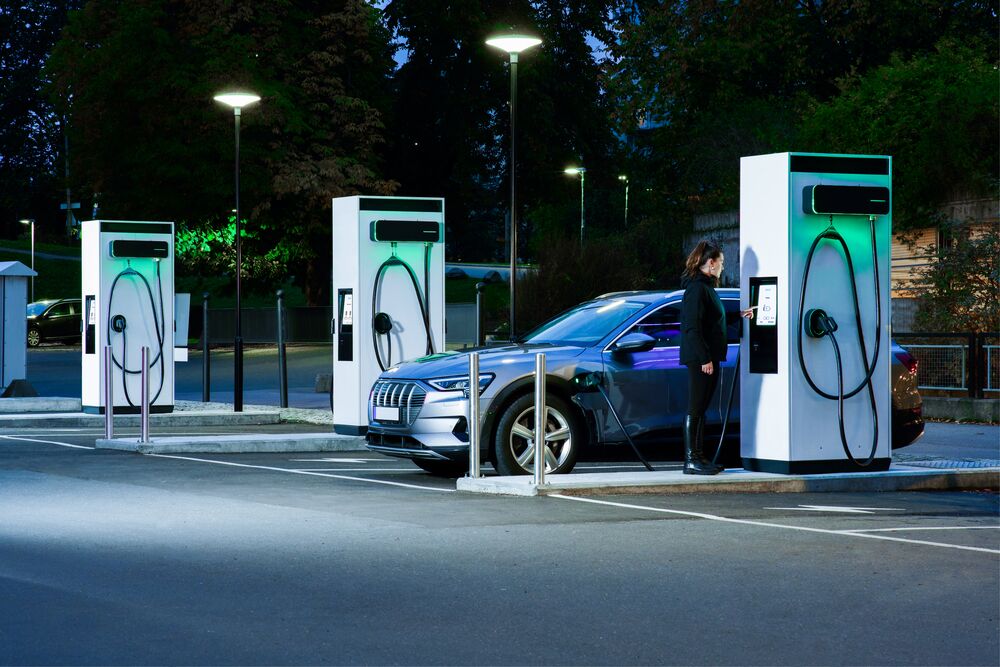The image depicts a nighttime scene at an electric vehicle (EV) charging station with three towering, rectangular white EV chargers spaced apart. Each charger features black cabling with a charger plug, and a prominent black rectangular box at the top that glows green. A woman with long brown hair tied in a ponytail, dressed in black leggings, a black jacket, and tall, shiny black boots, is operating the touchscreen on the charger, likely to charge her vehicle. Her silver-gray SUV, potentially an Audi with silver rims, is plugged into one of the chargers. The SUV appears to have minor damage on the right side near the wheel. The scene is set against a backdrop of tall bushes and pine trees, and is illuminated by several tall light posts scattered around the area.